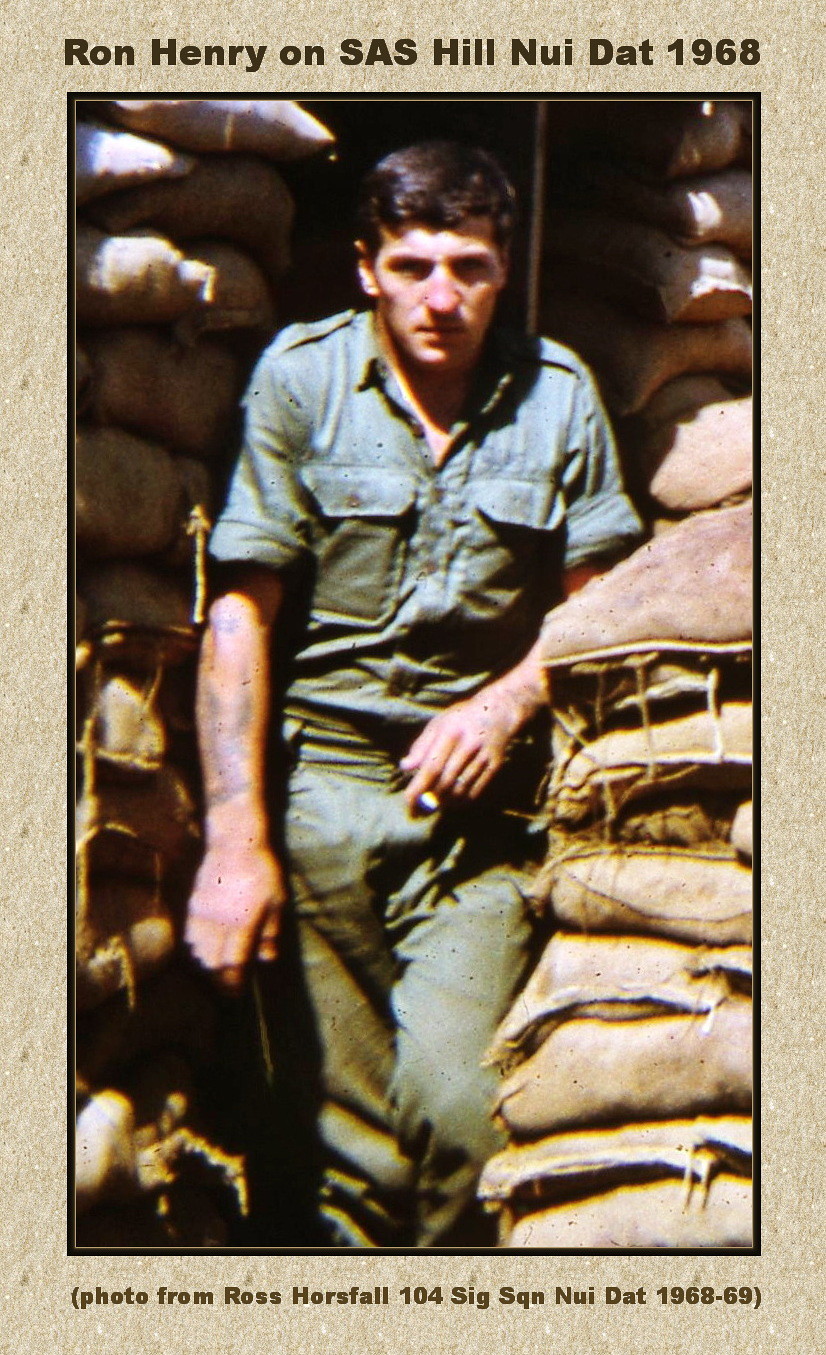The photograph depicts a soldier named Ron Henry, as indicated by the text above the image, "Ron Henry on S.A.S. Hill, Nui Dat, 1968." The soldier is a white man with short black hair, captured in between stacked sandbags, creating a fortified backdrop. His uniform consists of a green button-down shirt with two breast pockets and matching green khaki pants, cementing the military context. His left arm is casually propped up on a sandbag, while his right arm, displaying a tattoo, hangs by his side. The image has a slightly sepia-toned, aged appearance, with the background exhibiting a granulated brownish-gray color. Ron Henry gazes intensely at the camera, his expression a mix of sadness and mild anger. Below the photograph, there is a smaller caption stating, "Photo from Ross Horsfall, 104 SIG SQN, Nui Dat, 1968-69."